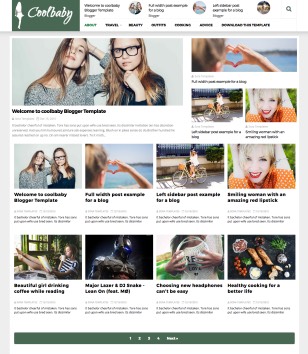The image features a stylish and dynamic webpage titled "Cool Baby." The design prominently displays white text stating "Cool Baby" and includes the white outline of a person. The webpage is structured into various sections such as "About," "Travel," "Beauty," among others, each showcasing a range of vibrant images. The main content appears to revolve around blog posts authored by two women, one of whom wears glasses and both possess long brown hair, discussing diverse topics.

Key visuals include:
- A blog section, richly illustrated with images related to the respective posts.
- A food-related image showcasing potatoes alongside cherries, promoting healthy eating.
- A close-up of a person holding headphones, potentially discussing audio gear or music.
- An image featuring a superhero character dressed in a gray uniform.
- A serene scene of an individual sitting on a porch with their feet up, engrossed in a book.
- A photo of someone sitting next to a bicycle, evoking themes of outdoor activities or travel.
- A heartwarming visual of a person forming a heart shape with their hands against a watery backdrop, symbolizing love or mindfulness.

The overall design maintains a clean, white background, punctuated by various blog posts and unified by green accent colors at the top and bottom, creating a crisp, engaging appearance.